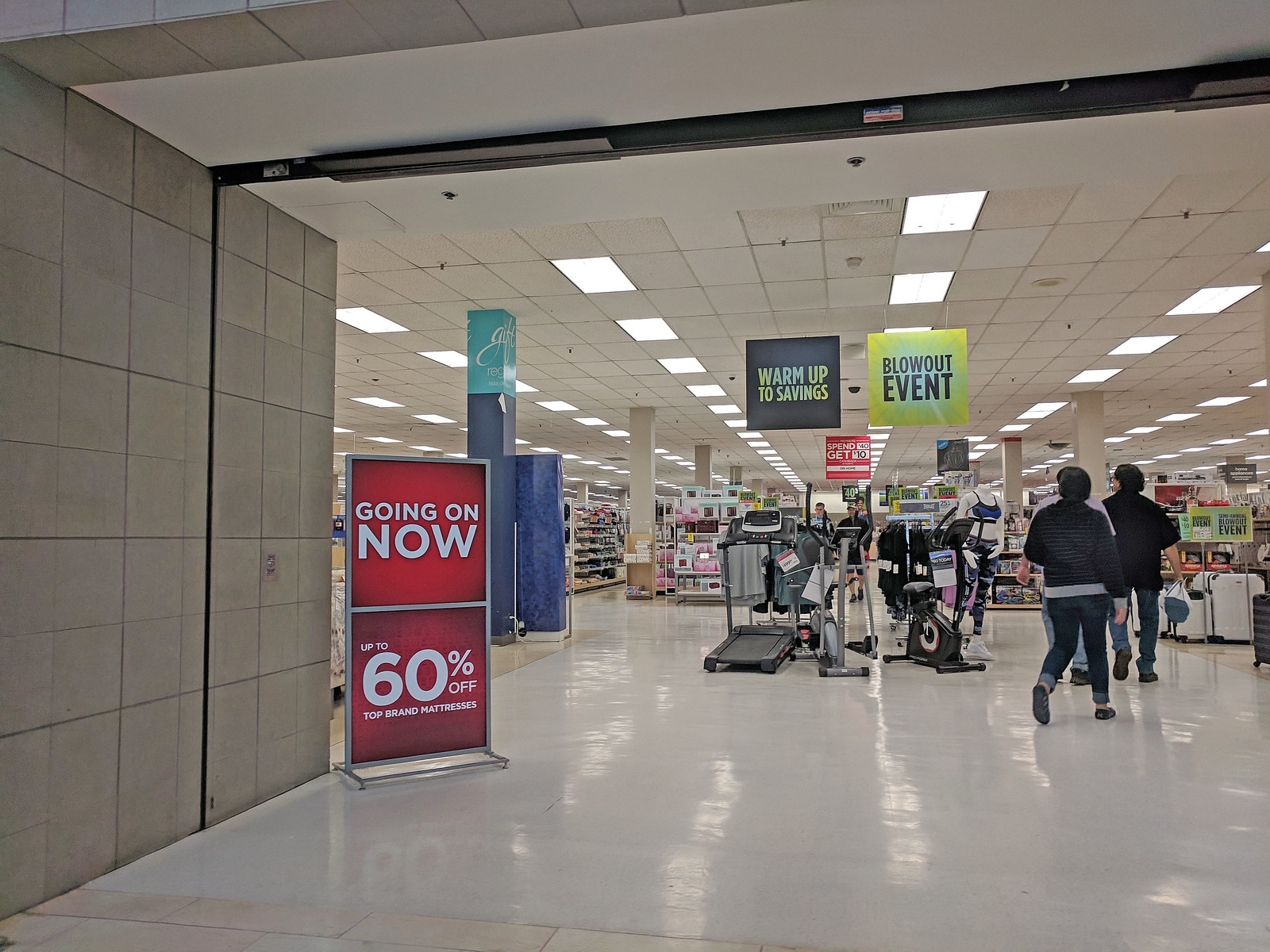The image depicts the interior of a large commercial building, likely a builder's merchant or similar wholesale retailer, characterized by its minimalist industrial aesthetic. The environment features a grey color palette, with the floor, ceiling, and walls all in shades of grey. Overhead lights stretch into the distance, creating a long perspective. In the foreground, two figures dressed in dark hooded clothing walk away from the camera, their forms adding a sense of scale and human presence to the expansive space.

Prominently displayed on the left side is a bold red sign with white text that reads "Going Now 60% Off." Near the shopping trolleys, there is a bright yellow sign announcing a "Blowout Event," emphasizing significant sales or discounts available within the store. Adjacent to this is a grey sign that invites customers to "Warm Up to Savings." Various other signs are strategically placed throughout the space, advertising different products and enticing shoppers with their offers. The overall scene suggests a promotional event, with multiple signs aimed at attracting customer attention to significant savings and deals.